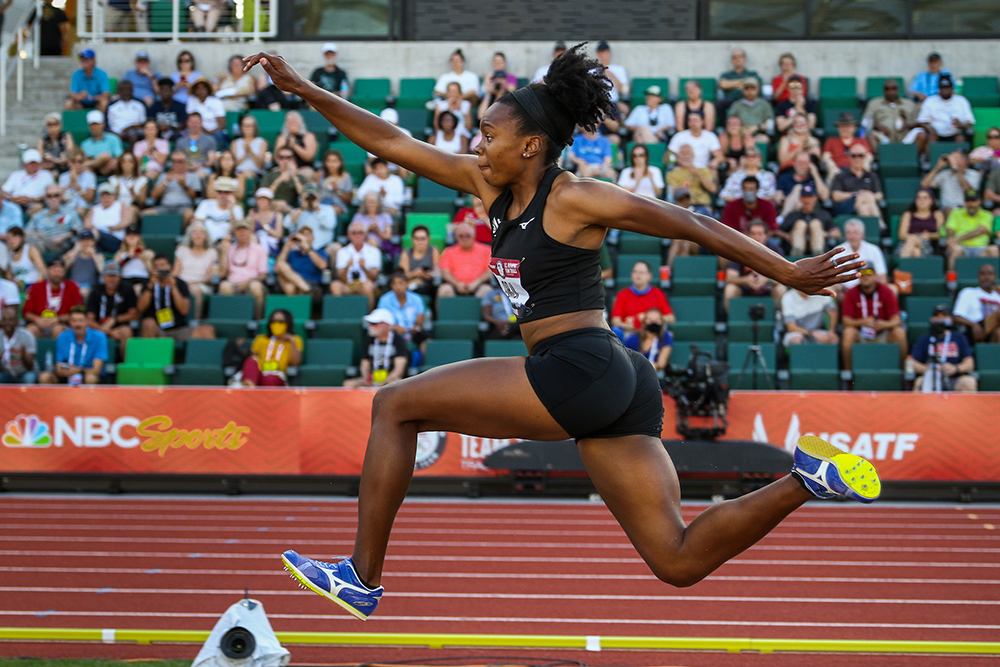This color photograph captures a high-speed moment during what appears to be a U.S. Track and Field event, possibly Olympic tryouts, featuring a black female athlete in motion. She is dressed in a black tank top, black shorts, and blue racing spikes with distinctive yellow soles. The spikes suggest a high-performance track competition, potentially a triple jump. The athlete, positioned at the center of the image, is airborne, showcasing her muscular build and intense focus. The red track she races on is marked with white and yellow lanes. The background reveals an orange NBC Sports banner with the NBC Peacock logo and a USATF (U.S. Track and Field) signage, indicating the event's prestigious nature. The stands filled with green seats are about half full with spectators, adding to the competitive atmosphere, while a television camera suggests live broadcasting of the event.